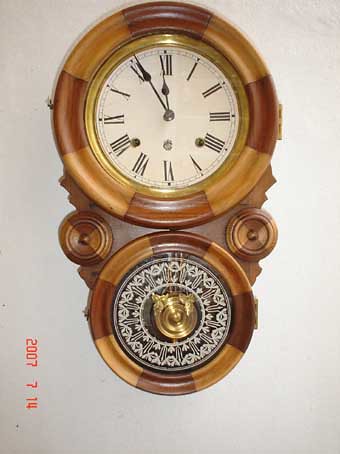A photograph taken on July 14, 2007, from inside a home features an intriguing and unique clock. The clock is constructed from two wooden circles connected by a central wooden piece. The upper circle serves as the clock face, adorned with Roman numerals from I to XII, all presented in an elegant Times New Roman font. The clock exhibits a refined set of hands—a delicate second hand, an hour hand, and a minute hand—precisely indicating the time at 12:56.

Embedded within the upper circle are two holes designed for cranking the clock when it needs winding. The bottom circle contains a pendulum, which swings rhythmically back and forth. This pendulum, crafted from golden material, is visible through a small glass window at the bottom of the clock. The glass itself is intricately etched with a decorative design, offering a beautiful view of the pendulum's movement. Both wooden circles showcase intricate inlaid patterns, with varying shades of wood that enhance the overall aesthetic. This clock is not just a timekeeper but also a piece of art, likely a cherished possession of its owner.